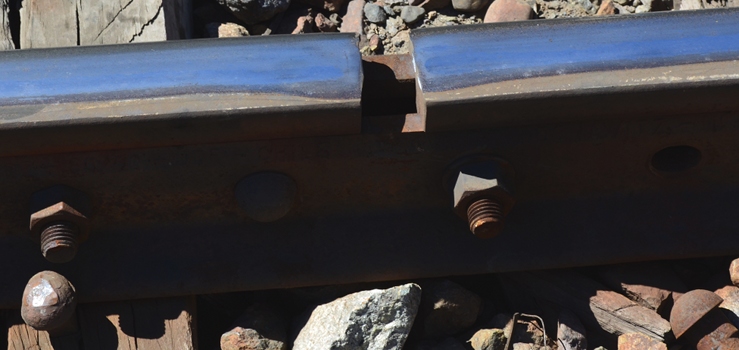This close-up image captures a section of an aged and possibly abandoned railroad track. The focus is on the various components that make up the track, revealing rusted nuts, bolts, and screws that suggest a long period of exposure to the elements. The steel rails, showing signs of wear, run parallel through the frame, while the wooden ties, placed horizontally, support the structure. Scattered between the wooden planks are numerous rocks and debris, adding to the impression of neglect. The overall condition of the track, coupled with the rust and debris, indicates that it may no longer be in active use or has been poorly maintained over time.